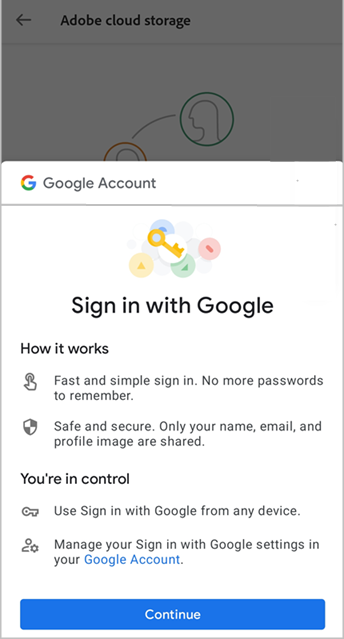The image displays a screenshot taken from a smartphone. At the top of the screen, the muted gray header reads "Adobe Cloud Storage," indicating the context of the pop-up overlay. Dominating the scene is a large white dialogue box where the text "Google Account" is prominently featured, accompanied by Google's iconic multicolored capital 'G.'

Beneath this, a golden key icon is encircled by small red, blue, yellow, and green circles, mirroring Google's color scheme. The phrase "Sign in with Google" is printed in bold black lettering. The text explains that this method provides fast and simple sign-in without the need to remember passwords.

Further down, a shield icon is captioned with "Safe and Secure," reassuring the user that only their name, email, and profile image are shared. Another section, featuring a key icon, underscores that signing in with Google can be done from any device. A silhouette of a person with a plus sign next to it denotes the ability to manage sign-in settings from the Google Account.

The pop-up concludes with a blue "Continue" button at the bottom, inviting the user to proceed with the sign-in process.